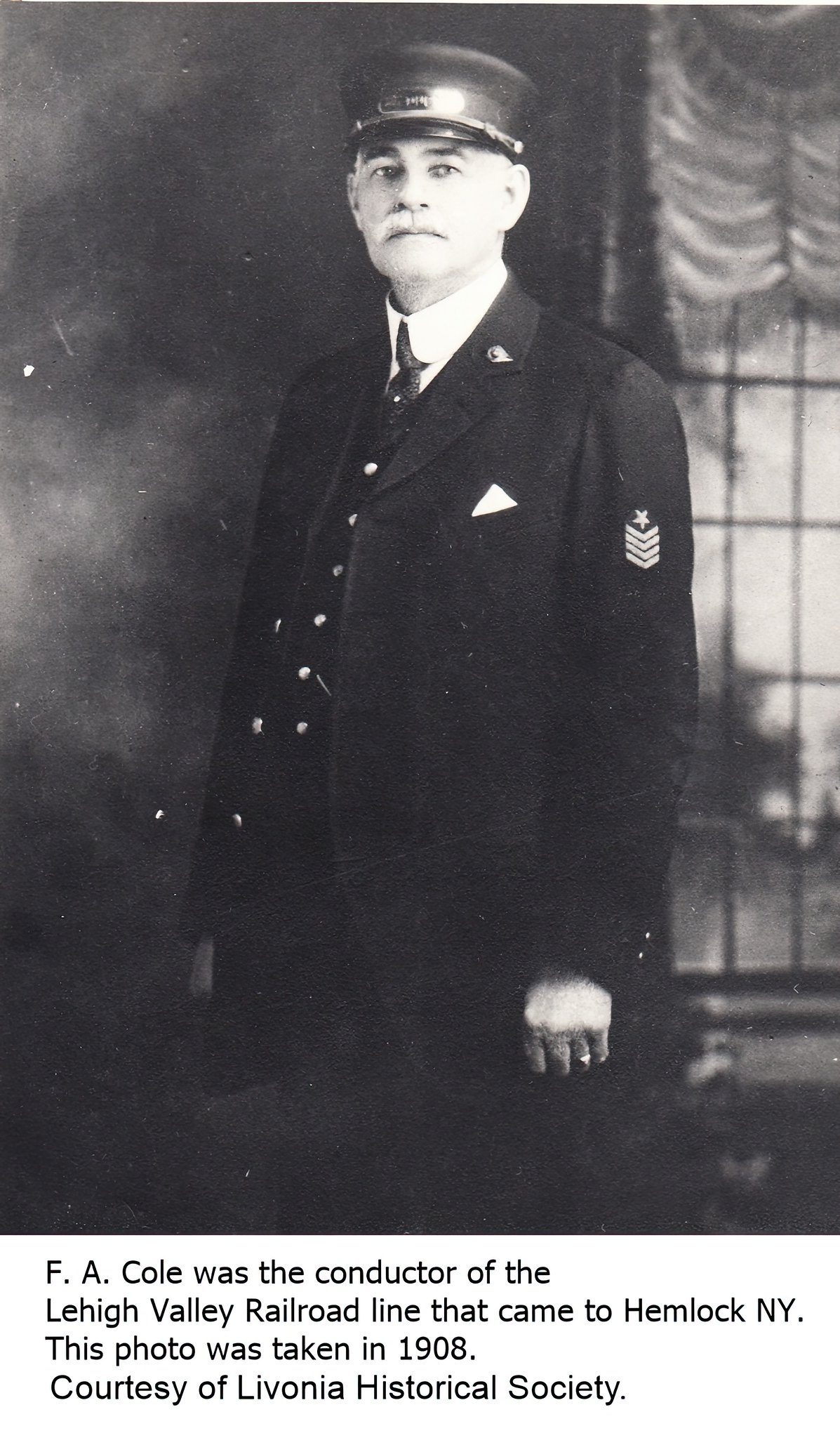This vintage black and white photograph from 1908, courtesy of the Livonia Historical Society, features F.A. Cole, the conductor of the Lehigh Valley Railroad line that serviced Hemlock, New York. The image captures an older man with a white mustache and light skin, standing in front of a window draped with curtains, with a faint view of a tree outside. Dressed in a distinguished uniform, Cole wears a black officer's hat with a small brim and engraving, a long black overcoat adorned with a pocket square, a tie, and a button-down vest. Notably, his jacket displays rank indicators on his left shoulder, including stars and stripes, and he also sports a lapel pin and a wedding ring. The photograph, clearly aged and distressed in some spots, immortalizes Cole in his authoritative role as a railroad conductor.